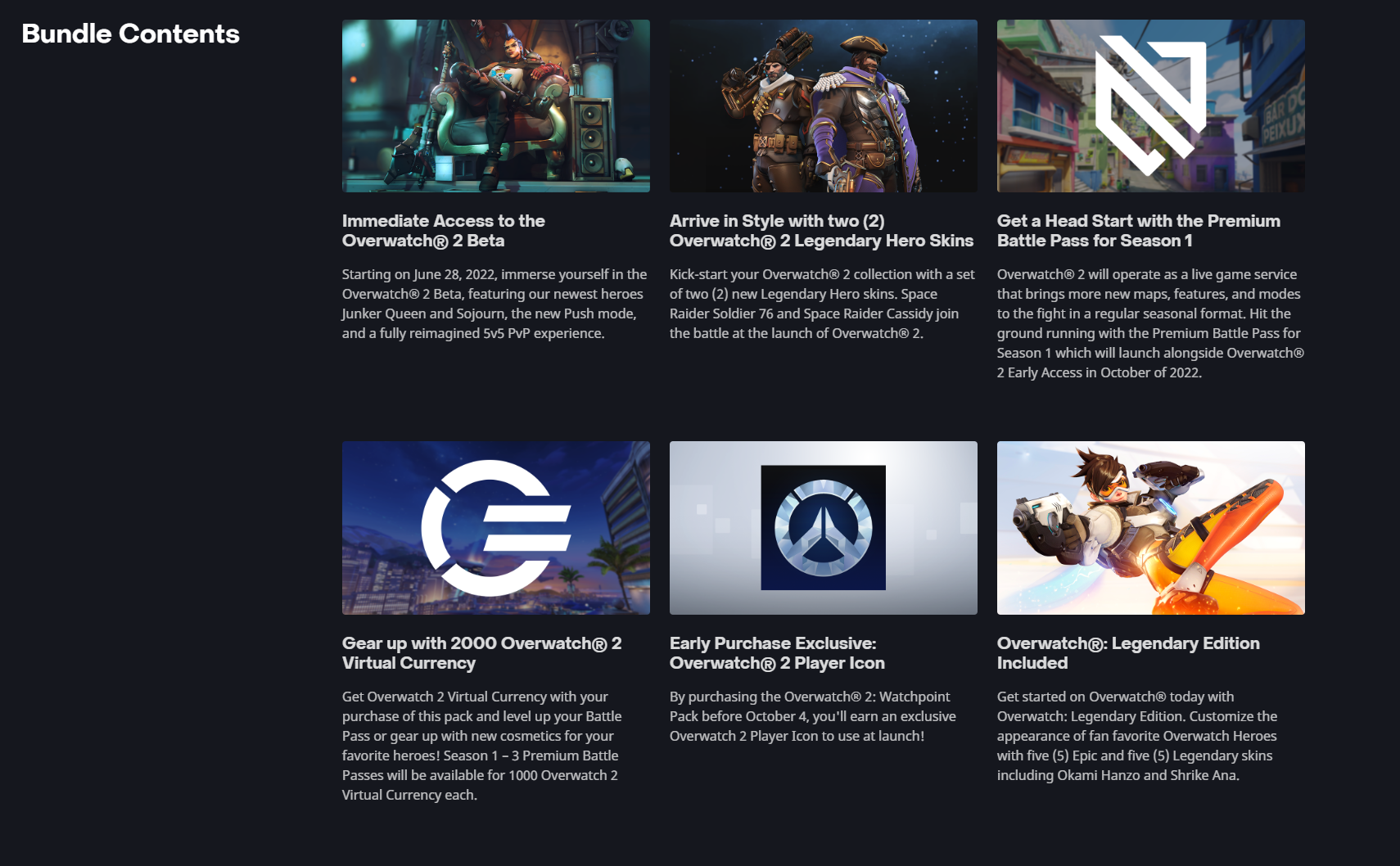The image features a promotional page for a bundle, set against an entirely black background. At the top, the title "Bundle Contents" is prominently displayed in white text. The layout is organized into sections, starting from the left and moving to the right.

On the left side, there is a section promoting "Immediate Access to the Overwatch 2 Beta," accompanied by an image of a game character seated in a room. To the right of this, the caption "Arrive in Style with Two Legendary Hero Skins" is displayed next to an image of two game characters standing together.

Further to the right, another segment showcases an emblem in white, with the text "Get a Head Start with the Premium Battle Pass for Season One." Below this, additional text reads "Gear Up with 2000 Overwatch 2 Virtual Currency," highlighting the bonus virtual currency available with the purchase of this bundle. The text goes on to explain that the currency can be used to level up the battle pass or acquire new cosmetics.

Towards the bottom of the page, more content sections are visible to the right, although the details are not fully captured in the image. The overall design is sleek and cohesive, providing a comprehensive overview of the contents included in the bundle.